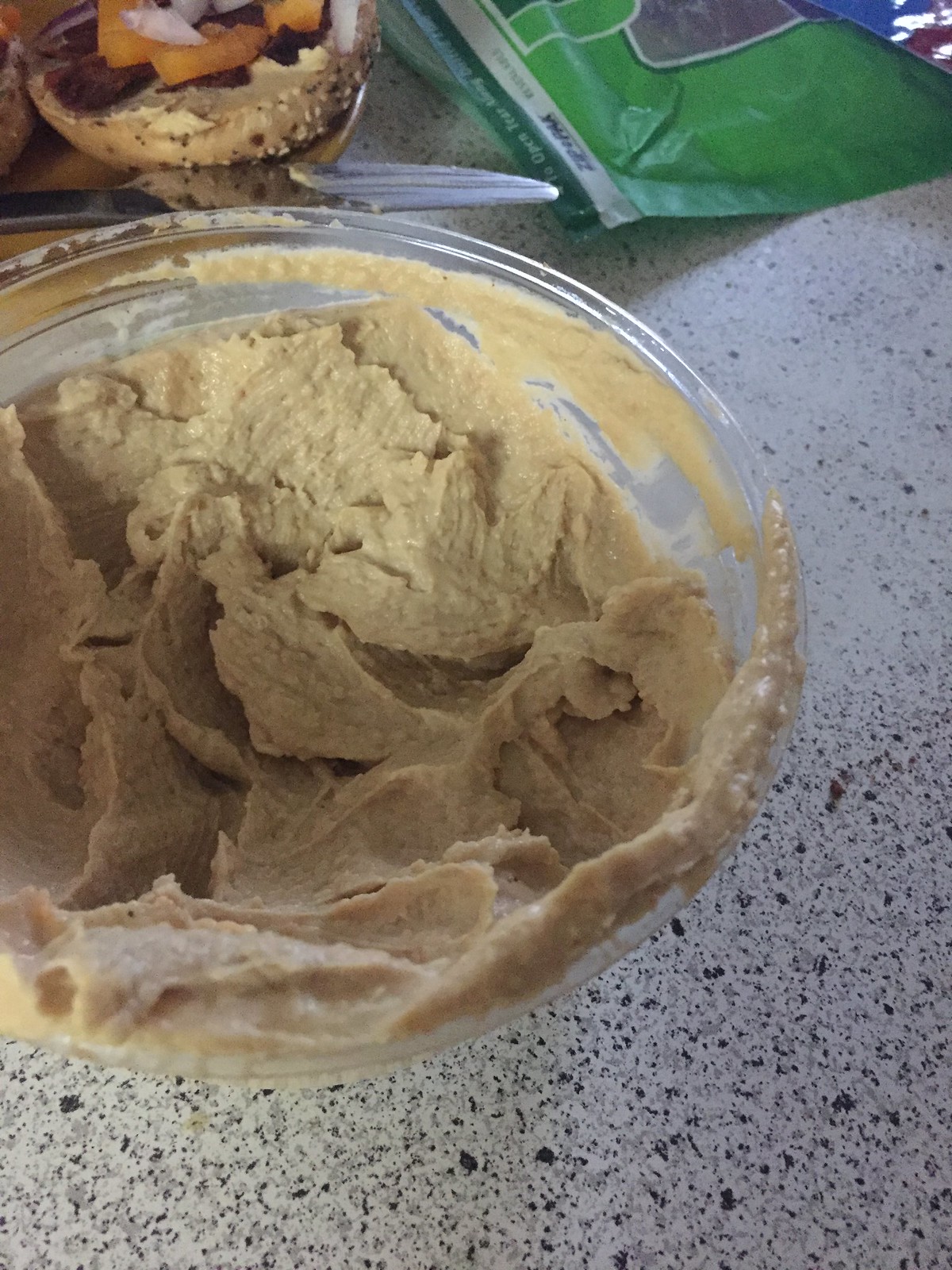This photograph features a thick, creamy beige hummus spread, partially filling a clear round plastic container that occupies the majority of the image. The hummus has a smooth texture but clings to the sides, showing evidence of having been dipped into several times. This container sits on a white countertop with a terrazzo pattern of black and gray speckles, possibly granite. Toward the top of the photograph, there is a half-eaten sesame seed bagel smeared with some of the hummus and topped with chopped orange and purple vegetables. A butter knife, bearing some streaks of possibly residual butter, leans on an orange plate underneath the bagel. In the top right corner, a green, mostly empty packaging bag is partially visible.